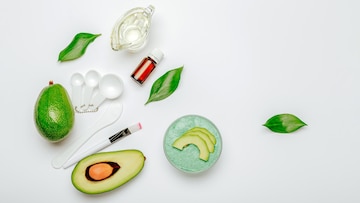The image displays a minimalist and professionally curated still life against a clean, gray background. At the center, there's a halved avocado with its pit intact, accompanied by another half nearby. Situated beside the avocado is a small greenish tray containing slices of avocado. To the right of these, there is a green leaf that adds a touch of nature to the composition. Below and slightly to the left of the avocado, a small blue plate holds what looks like chopped pieces, possibly pineapple or more avocado slices. In the upper portion of the image, a green fruit with a stem is visible, likely a lime. Scattered around, there are three white plastic measuring scoops of varying sizes and a brown bottle with a dropper top. Near the top center, a green leaf and a vial with a white cap, tinged with green hues, add to the assortment. The entire arrangement gives a sense of organized randomness, likely intended to showcase these items in a clean, aesthetically pleasing manner, possibly for a website or product photography project.